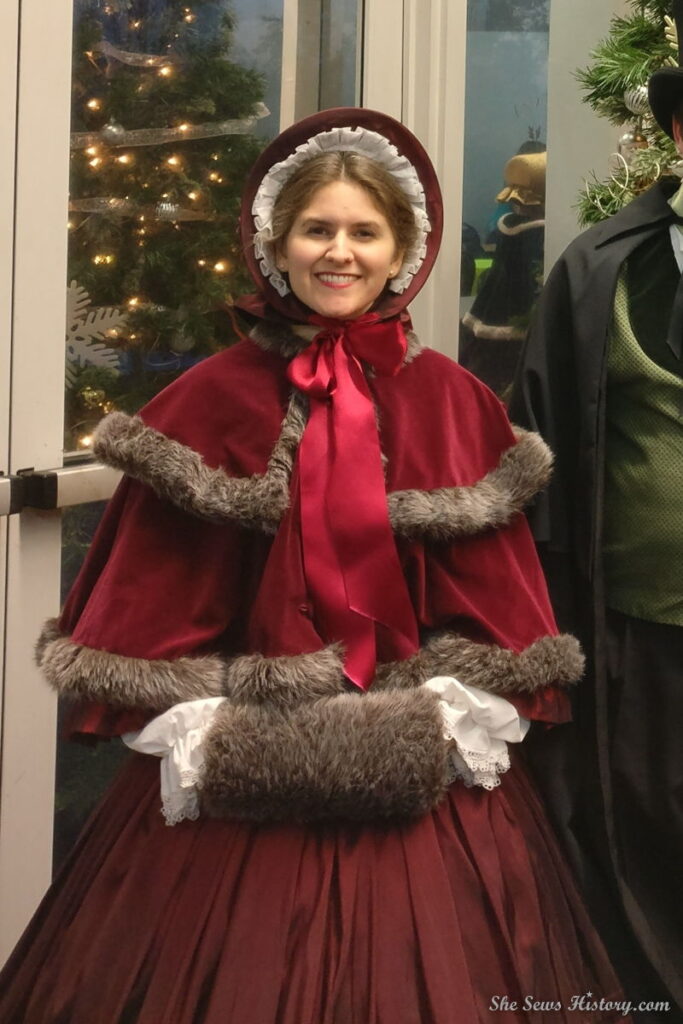In this detailed photograph, a woman is dressed in an elaborate, festive, Victorian-style outfit that evokes the holiday spirit. The image features a close-up of her smiling face, framed by a red bonnet adorned with white lace underneath. Her long brown hair is mostly obscured by the bonnet, and she wears pink lipstick that complements her cheerful expression. The ensemble includes a red coat, possibly velvet on the torso, lined with brown fur that matches her brown fur muff where she keeps her hands warm. Her petticoat is a darker, maroon shade of red, contrasting with the bright red velvet of her coat and the colossal, vibrant red ribbon tied in a bow at her neck. 

She stands in front of a modern door with a metal frame and glass panes, through which a lit Christmas tree and decorative snowflake are visible, enhancing the festive atmosphere. The door features a metal bar handle, reinforcing the contemporary setting. On the right edge of the photograph, partially cut off, a man is visible wearing a black brimmed hat, a black cape, a green vest, and black pants, complementing the historical theme.

At the bottom right corner of the image, the text "shesewshistory.com" is displayed, indicating the source or theme related to historical dressmaking. The overall scene combines elements of the past with modern touches, creating a picturesque representation of holiday cheer.